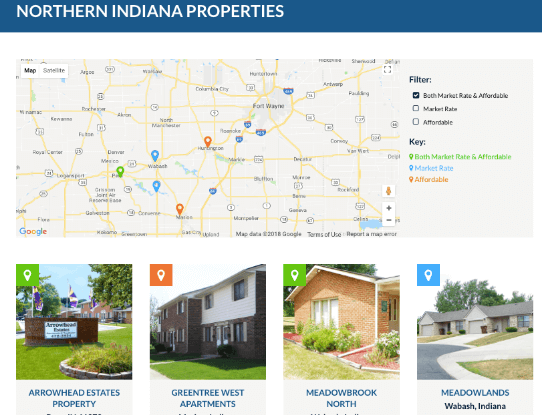The image displays a web page showcasing various apartment and housing units in Northern Indiana. At the top of the page, a blue header prominently features the text "Northern Indiana Properties" in bold white lettering. Below the header, on the left side, is an interactive Google map. Adjacent to the map, on the right side, is a vertical column of filters labeled "Market Rate and Affordable," with color-coded indicators: green for "Both Market Rate and Affordable," blue for "Market Rate," and orange for "Affordable."

The map itself includes detailed elements such as interstate highways, depicted as yellow lines, along with typical Google map functionalities like Street View and zoom controls (+/-). Below the map, four distinct property listings are displayed, each marked with a corresponding color code from the key.

1. **Arrowhead Estates Property**: Represented with a green marker, featuring a photograph of the property's entrance sign.
2. **Green Tree West Apartments**: Indicated with an orange marker, showing a picture of the apartment buildings' front facade.
3. **Meadowbrook North**: Highlighted with a green marker, illustrated with a photograph capturing a garden and the side of an apartment complex.
4. **Meadowlands**: Marked with a blue marker, accompanied by an image of a residential home with two garages, located in Wabash, Indiana. 

Each property provides a visual reference through the photographs and color codes, helping users easily identify the type and location of the housing units available.